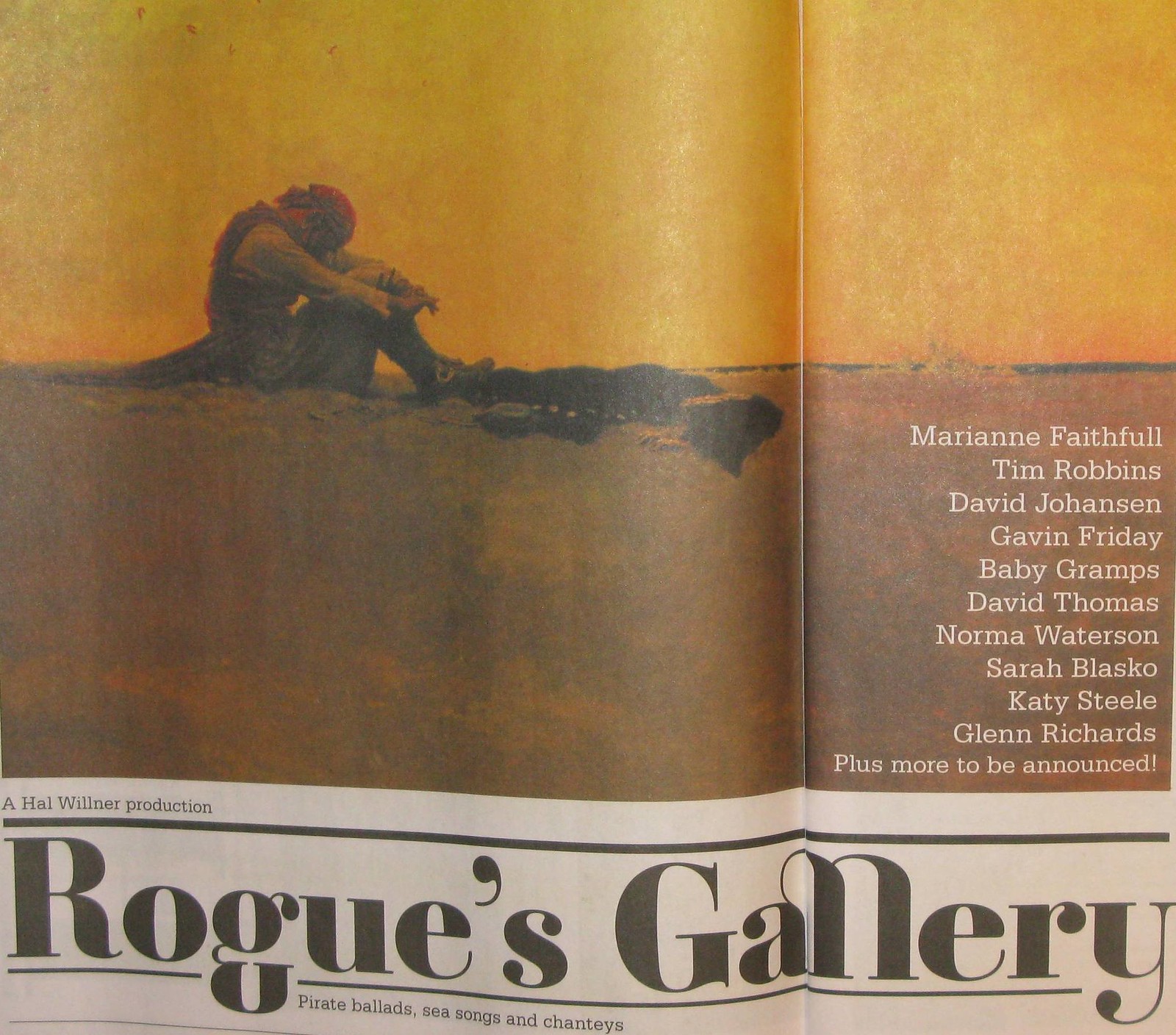The image is an evocative scene that appears to be the cover of a record album or a newspaper, featuring a solitary pirate seated on a sandy beach. The upper portion of the image, set against a faded yellow and dark brown background, showcases the pirate character dressed in a red bandana, a brown vest, and a gray long-sleeved shirt. His head is bowed, and his arms are resting on his knees as he gazes down at the sand. To the right of the pirate, in the bottom-right corner, white text lists the names: Marianne Faithful, Tim Robbins, David Johansson, Gavin Friday, Baby Gramps, David Thomas, Norma Watterson, Sarah Blasco, Katie Steele, and Glenn Richards, with a note indicating more names to be announced. The lower portion of the image, set against a whitish-gray background, prominently features the title "Rogues Gallery" in large black letters, followed by the subtitle "Pirate Ballads, Sea Songs, and Shanties" in smaller print, denoting it as a Hal Wilmer production. The overall composition blends elements of melancholy and nostalgia, capturing the essence of maritime lore and pirate balladry.